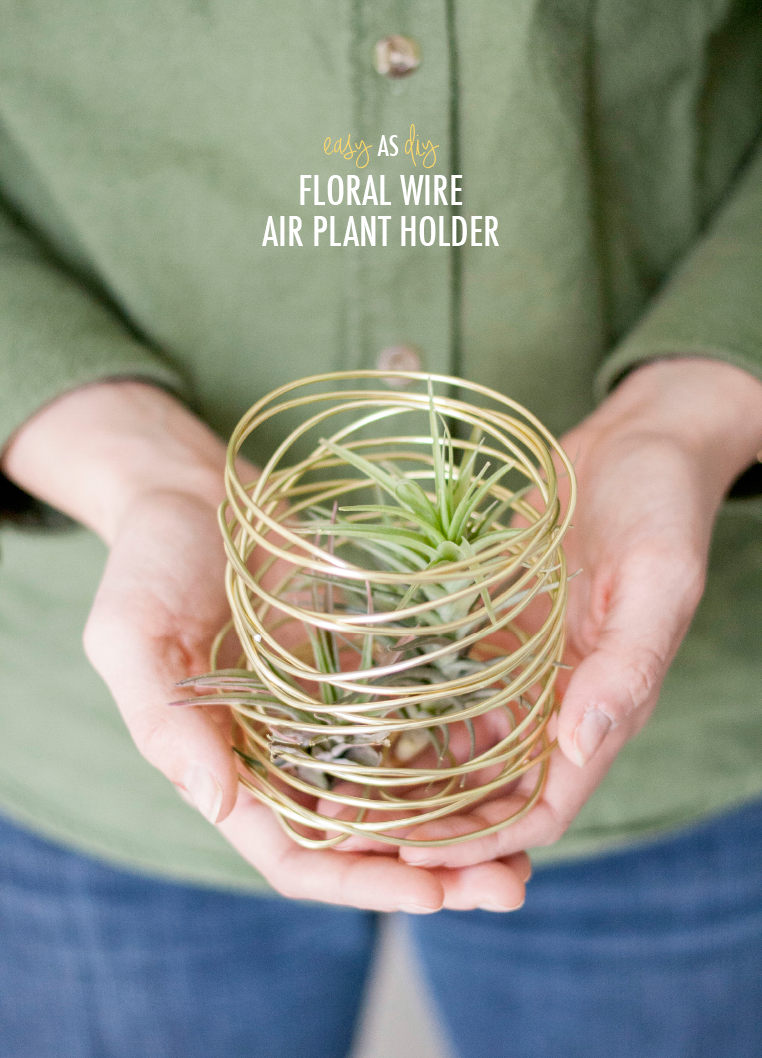The image features a person, likely a woman given the long fingernails, dressed in a thick, long-sleeved, green button-down shirt and blue denim pants. The shot is framed from the upper thighs to the torso, emphasizing the hands, which are cupped together in front of her. She is holding a gold, cylindrical, spring-like structure made from twine, which serves as a DIY floral wire air plant holder. Inside this holder, there are a couple of small, green, desert-looking plants with long, narrow leaves, just starting to sprout. The main focus of the image is on the plant holder and the small plants, with text at the top reading "Easy as DIY Floral Wire Air Plant Holder." The person's shirt features brownish buttons, adding a subtle detail to the overall composition.